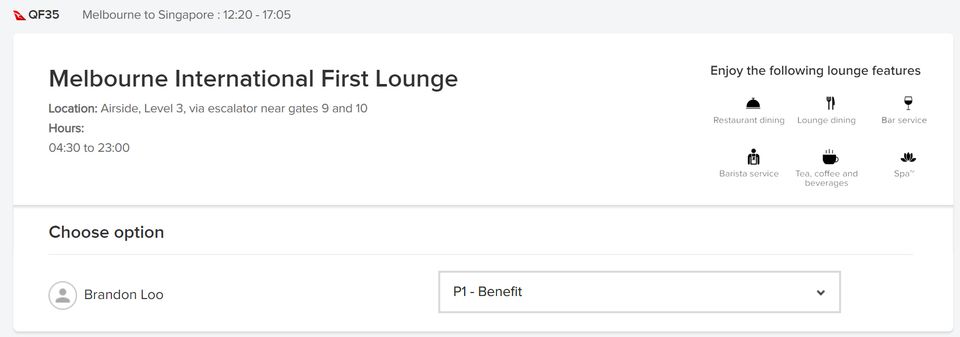The image features a grey-bordered panel, wider at the top, displaying the following information:

At the top center, in bold lettering, it reads "QF 35 Melbourne Singapore 1220-1705." Beneath this, a prominent white box contains the text "Melbourne International First Lounge" in large black letters. Below this headline, smaller text provides additional details: "Location: airside, Level 3 via escalator near gates 9 and 10. Hours: 0430 to 2300."

On the right side of the panel, a section lists the lounge's amenities, stating, "Enjoy the following lounge features: restaurant dining, lounge dining, bar service, barista service, tea, coffee, and beverages, and spa."

Lower on the panel, there is another, smaller box with the text "Choose Option," followed by a dividing line. Below this is a generic default profile picture with the name "Brandon Lou" next to it. To the right, a dropdown menu box displays the text "P1 - Benefit."